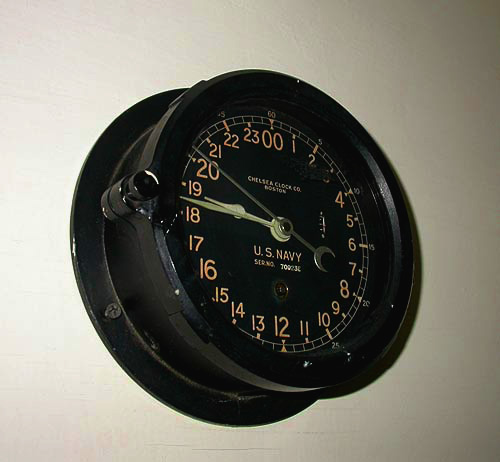A square image features a tan or light brown background, showcasing a vintage clock or gauge removed from a U.S. Navy vessel. The clock, which is predominantly black, has a circular metal bezel face adorned with knobs and is mounted onto a round base affixed to the wall with screws. Yellowish-orange numbers circle the clock face, ranging from 00 to 23. The timekeeping elements include white hour and minute hands, and a black second hand with a crescent moon tip. The displayed time reads approximately between 18:30 and 19:00 hours.